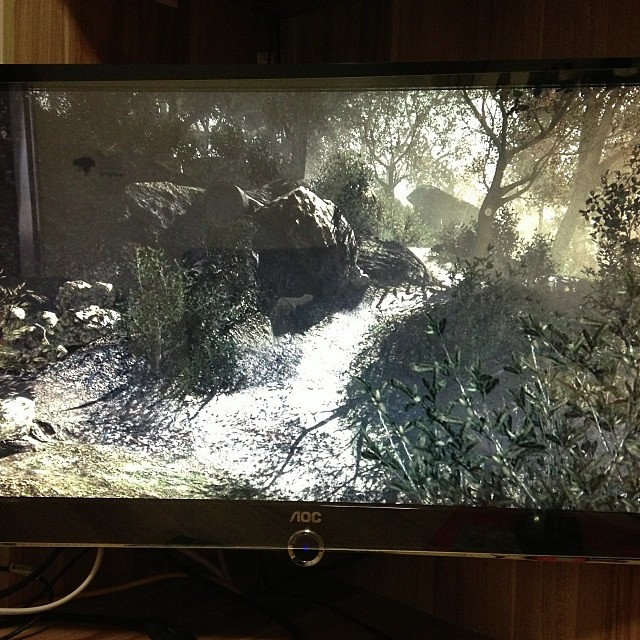The image depicts a computer monitor with a thin black border at the top and a wider black border at the bottom, featuring a silver trim and the branding "AOC" prominently displayed at the center bottom. The monitor is set against a background of light brown wood paneling, with visible white and black wires running behind it. Displayed on the screen is a brightly lit forest scene with dark green foliage and bushes on the right. In the foreground, a dirt pathway winds through the center, flanked by large boulders and trees, their trunks and leaves bathed in sunlight. There appears to be a pronounced contrast to the image, giving it a stark look. Some elements might suggest the presence of structures like rooftops in the distant background, though it’s difficult to distinguish clearly amidst the forest scape.